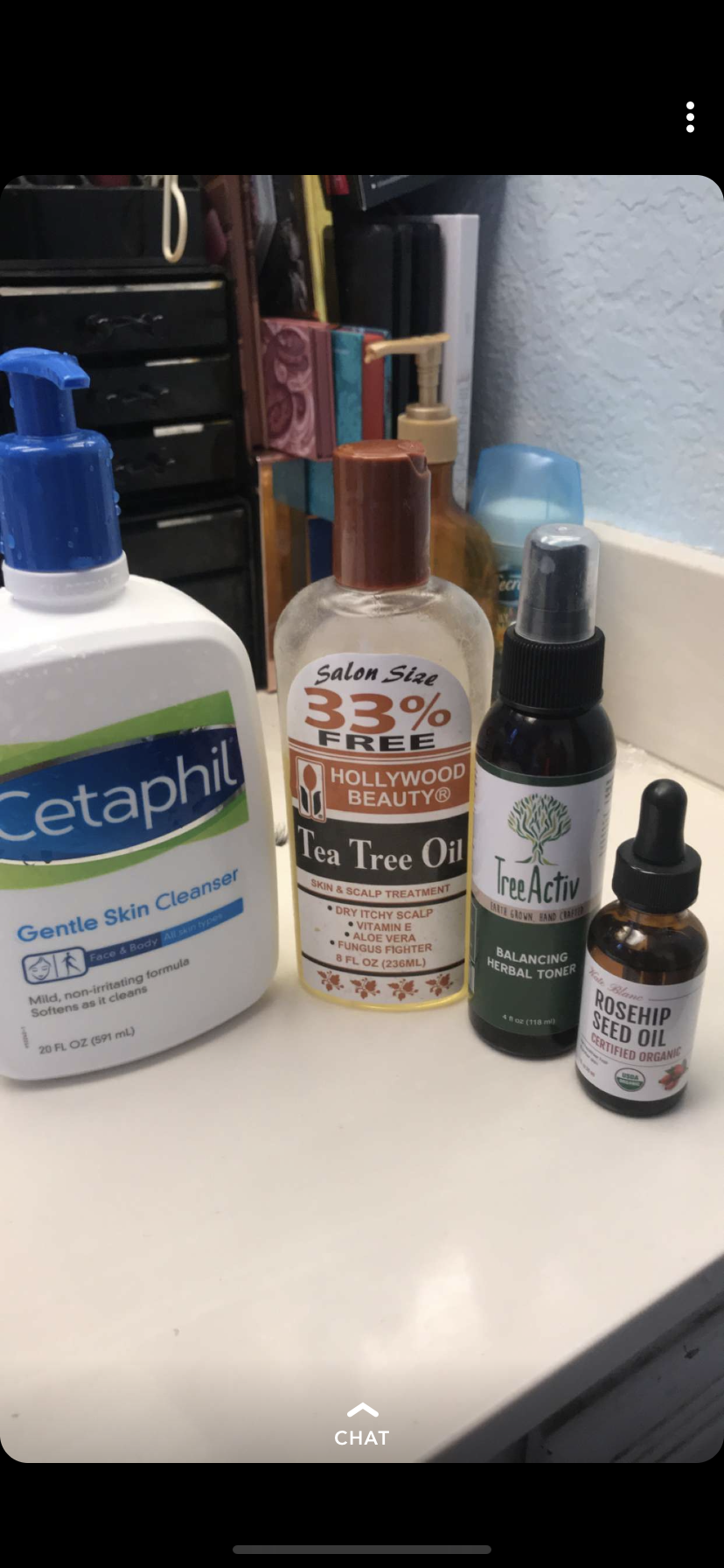This is a photograph resembling a screenshot taken on a phone. The top and bottom edges of the image are black, and a thin gray line is visible at the very bottom, while a small dot is present towards the top right corner of the black margin. At the bottom of the photograph, the word "CHAT" is displayed in white text.

The main focus of the image is a white countertop featuring four distinct bottles. Starting from the right, there is a small brown bottle with a matching brown cap. Next to it is a black bottle adorned with a white label, followed by a plastic bottle with a brown lid and a white label, identified as tea tree oil. The leftmost bottle is white with a blue pump lid.

In the background, sitting on the same countertop, there is a black drawer unit. Positioned to the right of this unit is a blue deodorant stick, another pump bottle, and several unidentified items standing upright in the corner. The wall behind the countertop is a very pale blue shade.